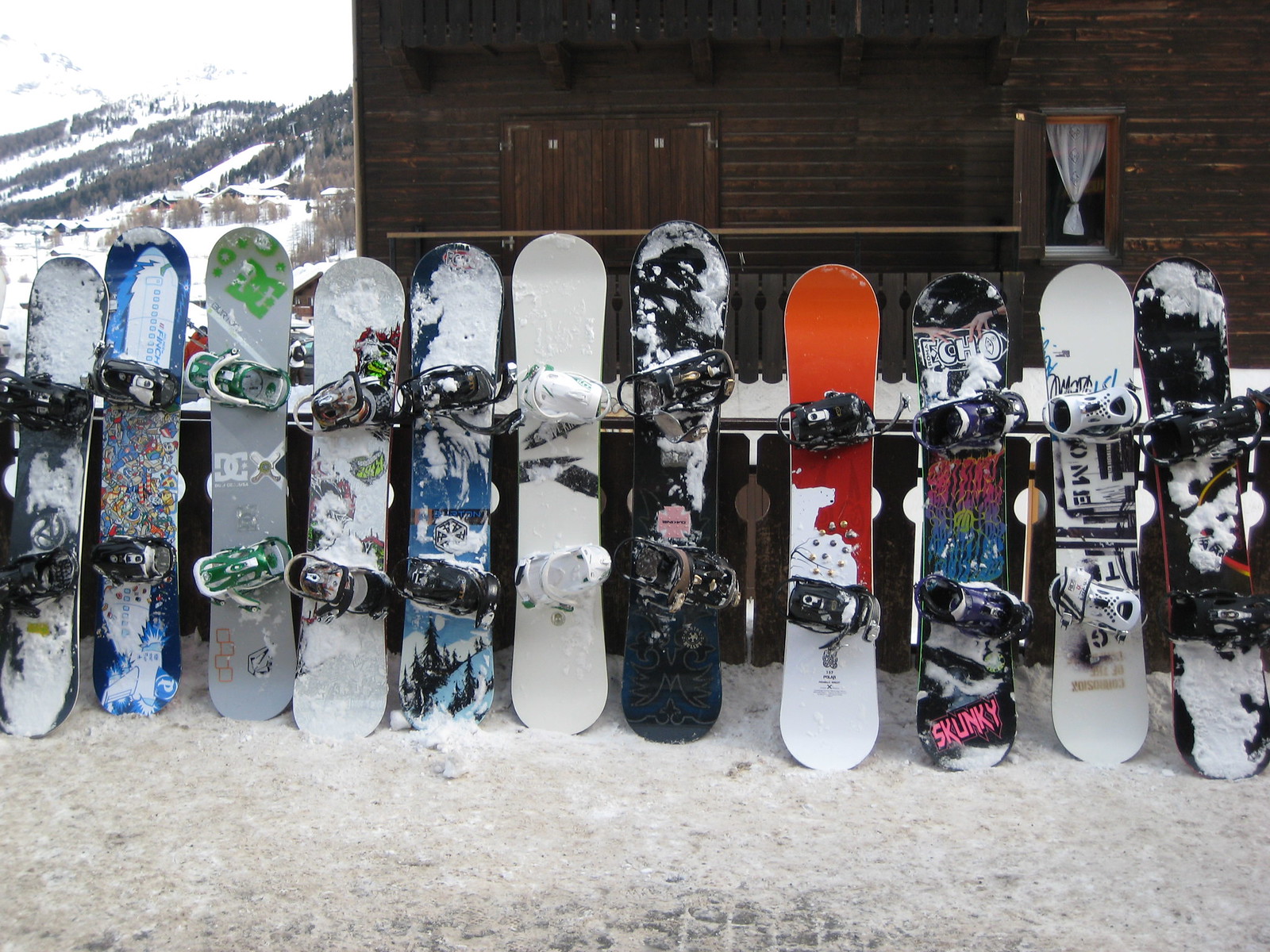This photograph captures a row of approximately 11 diverse snowboards standing upright against a wooden fence at a ski resort. The snowboards, varying in colors from white, black, orange, blue, green, to red, display an array of graphics, though many are heavily coated with snow, obscuring some details. They range in sizes and shapes, reflecting different users' preferences. The scene is set with a backdrop of a rustic wooden cabin with a window sporting a white curtain, nestled amidst a snowy landscape. In the upper left and back right, towering mountain ranges are visible, dotted with pine trees and ski slopes. A brown and white snow-covered ground extends in front of the snowboards, adding to the wintry ambiance.